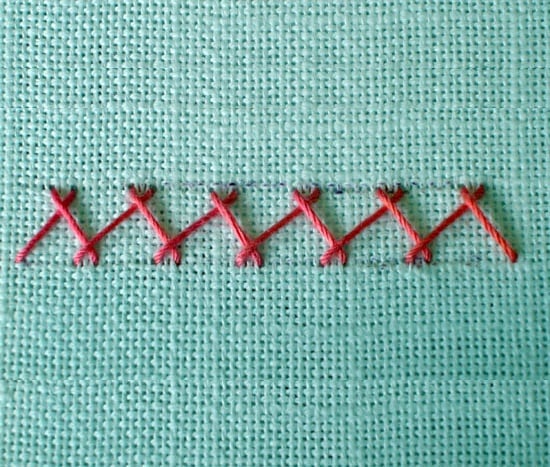This close-up photograph captures a square piece of light blue fabric with a discernible weave texture, reminiscent of a canvas or finely knitted material, punctuated by small holes. Dominating the center of the fabric is a series of six red stitches that span horizontally across the image. These stitches form shapes that can be described as teepees or pyramids, each consisting of two lines crossing slightly above the midpoint rather than at the center, resulting in a distinct crisscross pattern. The fabric fills the entire frame, showcasing its various shades of blue, influenced by the shadows and lighting, and lending the image an artistic, handcrafted feel.